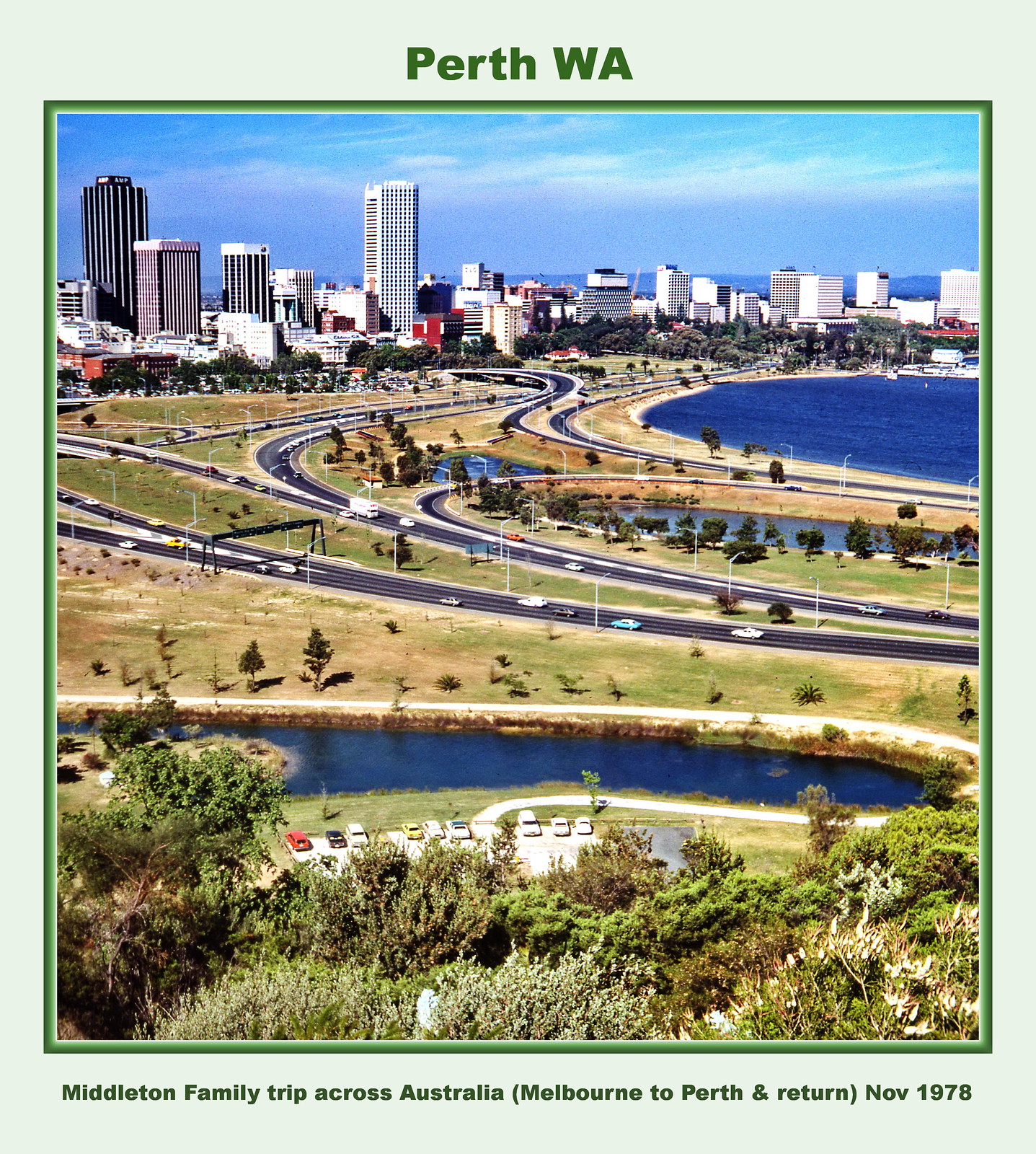The image is a card featuring a detailed photograph of Perth, WA. The card has a light gray border around the edges with green text indicating "Perth WA" at the top and "Middleton family trip across Australia – Melbourne to Perth return, November 1978" at the bottom. The central photograph is outlined with a dark green thin border inside a lighter green thicker one.

In the middle of the card is a sprawling cityscape of Perth, captured from an aerial perspective. At the top of the picture is a clear blue sky. Below it, the skyline of Perth features a mix of very tall buildings and medium-sized ones, with various colors including whites, blacks, and grays. To the right of the cityscape is a large body of water, likely a river or the ocean, which adds to the panoramic view of the city.

The middle of the image showcases a complex network of highways with multiple curvy, black paved roads running left to right and into the city. These roads are dotted with tiny cars, indicating the photo was taken from high above. Surrounding the highways are patches of green grasslands, and in the foreground, there’s another smaller water body, resembling a pond, with some grass, weeds, and shrubs nearby. The greenery, along with trees and shrubs, adds a natural frame to the busy urban and infrastructure scene.